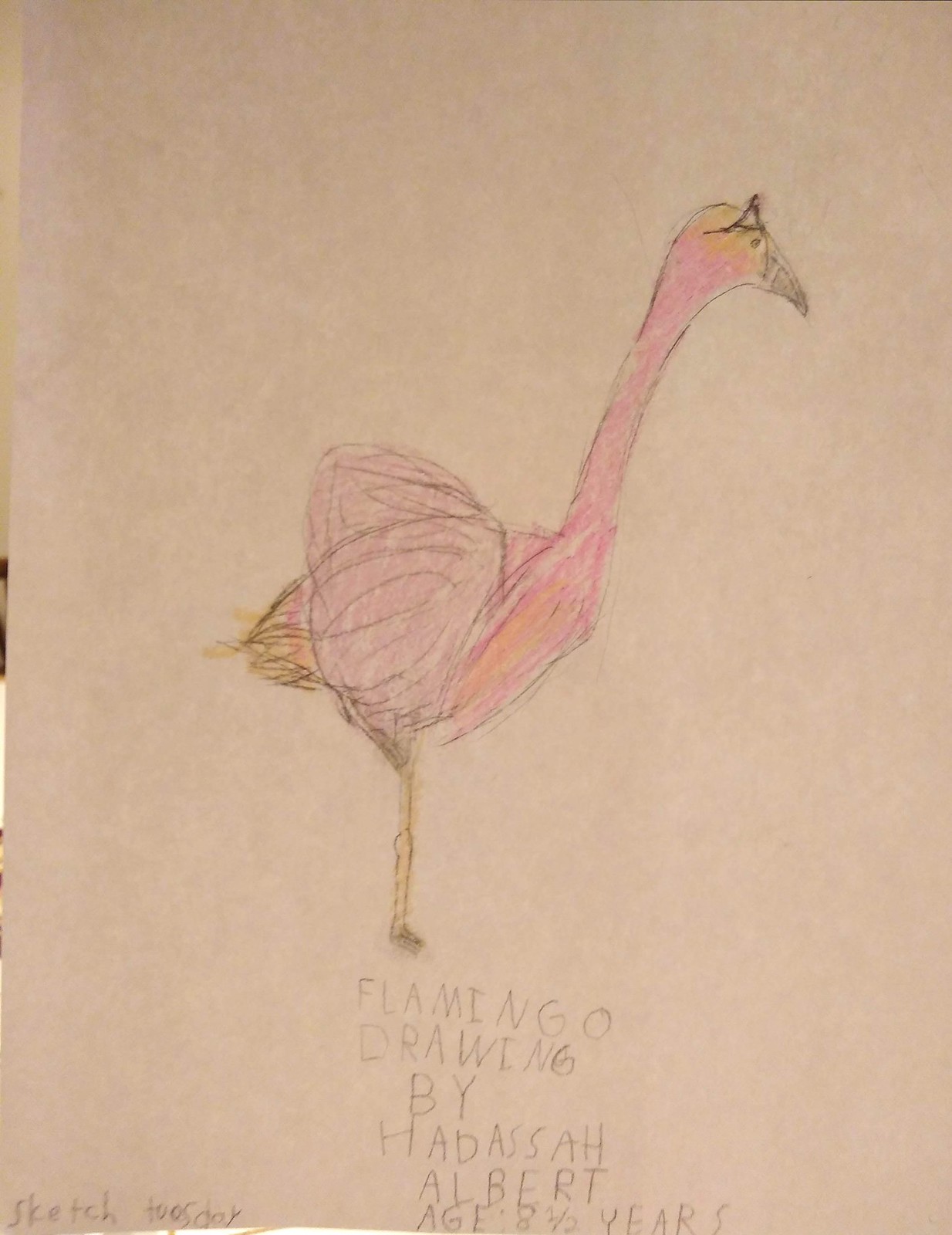This colored sketch depicts a whimsical flamingo standing in a side profile facing to the right. Though not highly detailed or photorealistic, the charm lies in its simplicity. The flamingo features a long, curved neck and a distinct black beak. Its fluffy wings are rendered in a soft pink, while hints of yellow accentuate the top of its head, underbelly, and tail. The bird stands on scrawny, thin legs, typical of a child's artistic interpretation. Below the sketch, a caption reads in capital letters: "FLAMINGO DRAWING BY HADASH ALBERT, AGE EIGHT AND A HALF YEARS." In the bottom left corner, another caption states: "Sketch Tuesday."